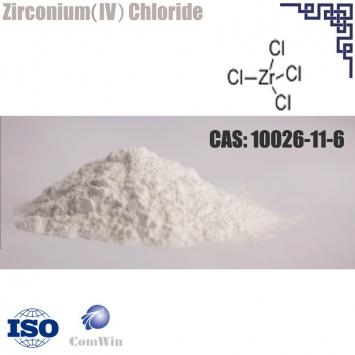The image depicts a scientific material related to zirconium chloride. At the top left corner, the text "Zirconium(IV) chloride" is displayed prominently on a white background. To its immediate right is a molecular diagram illustrating a zirconium atom bonded to four chlorine atoms. The upper right corner features a blue, curly design. In the center of the image, within a gray rectangular box, is a photograph of white powder set against a pink backdrop, identified as zirconium chloride. In the top right corner of this gray box, the chemical's CAS number "10026-11-6" is printed in black letters. At the bottom left, on a white background, is an ISO logo atop a globe image with longitude and latitude lines, while next to it is the word "ComWin" next to a sphere with a wing-like design emerging from the left. The ISO logo is blue, and the word "ComWin" is in gray.